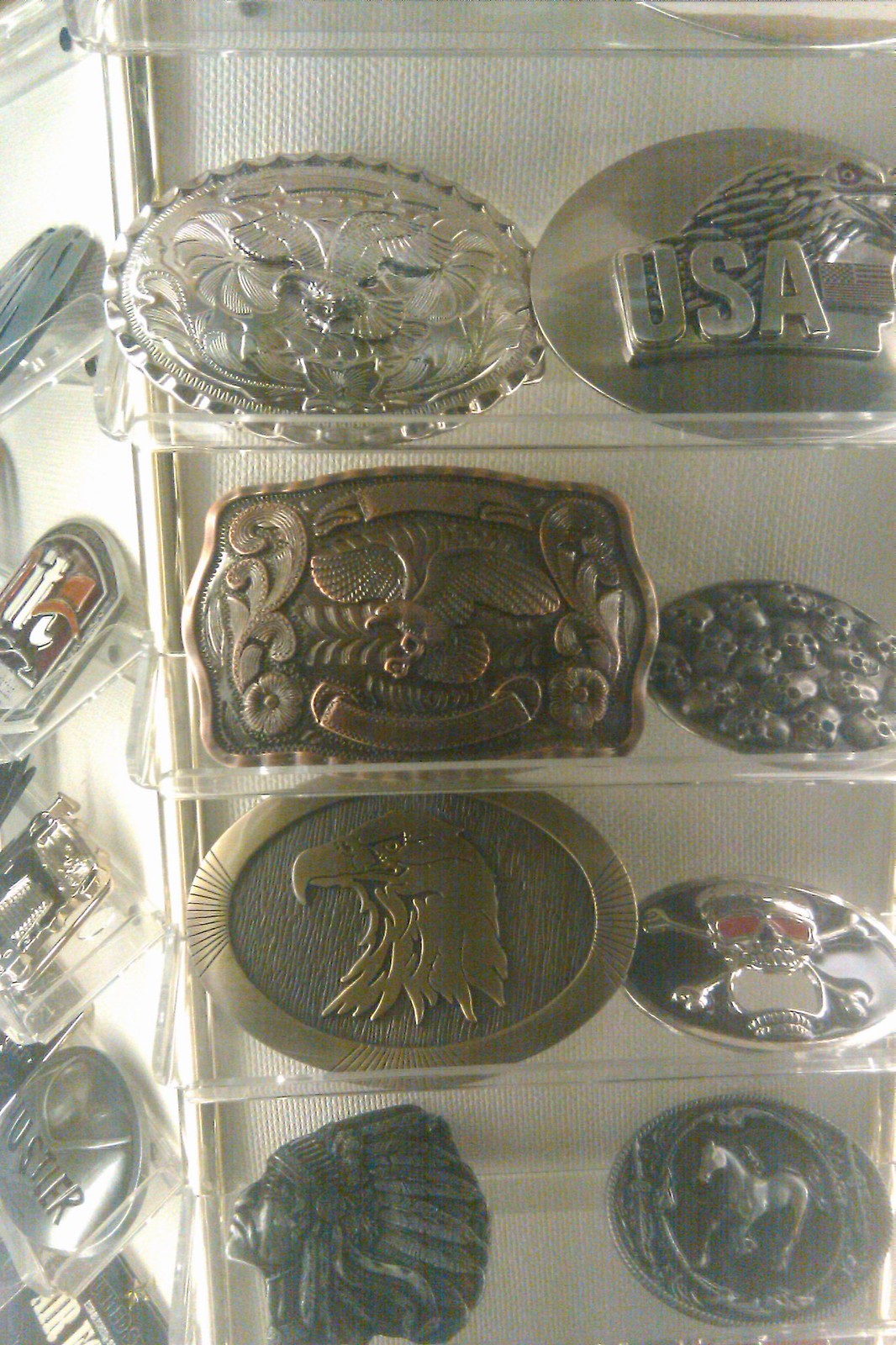This desaturated, color photograph features a collection of large, ornate belt buckles displayed on plastic shelves. The photograph captures four rows of these decorative buckles, each heavily embossed with intricate designs.

On the top shelf, to the left, there is a silver belt buckle adorned with an eagle design. Next to it, on the right, is another silver buckle featuring an eagle and the word "USA" inscribed on it. The second shelf houses a bronze buckle on the left that also appears to have an eagle motif, although it is less distinct. To its right, there is a smaller buckle decorated with circular patterns.

Descending to the third shelf, on the left, is a muted gold buckle with an eagle head facing left. Adjacent to it, on the right, is a buckle with a silver skull and crossbones, accentuated with red eyes. The bottom shelf displays a dark pewter buckle engraved with an Indian head in a full headdress, gazing upwards and to the left. To its right is another dark gray buckle featuring the image of a galloping horse.

The plastic shelving frames and supports these buckles, and the arrangement extends to the left side of the image, where the case turns a corner, revealing more of these embossed artifacts.